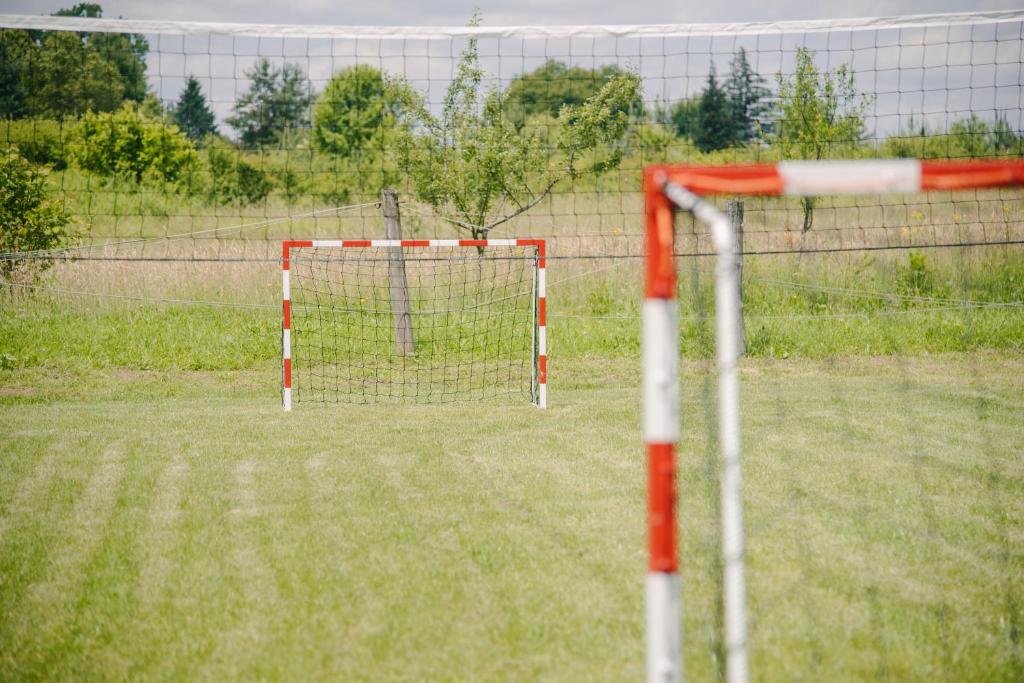This vivid photograph captures an amateur soccer field on a sunny day, spotlighting two small, orange and white-striped soccer goals. The closest goal features prominently in the foreground, partially visible, while the second goal stands fully in sight in the background, complete with its black net. The neatly mowed grass, adorned with visible lawnmower marks, stretches between the goals, indicating recent maintenance. Adding an intriguing detail to the scene, a volleyball net is strung through the middle of the goals. Further back, the field transitions into overgrown grass, which leads to a dense border of trees and shrubs, encapsulating the serene and undisturbed setting. The expansive blue skies overhead enhance this tranquil landscape where no one currently plays, underscoring a peaceful moment frozen in time.